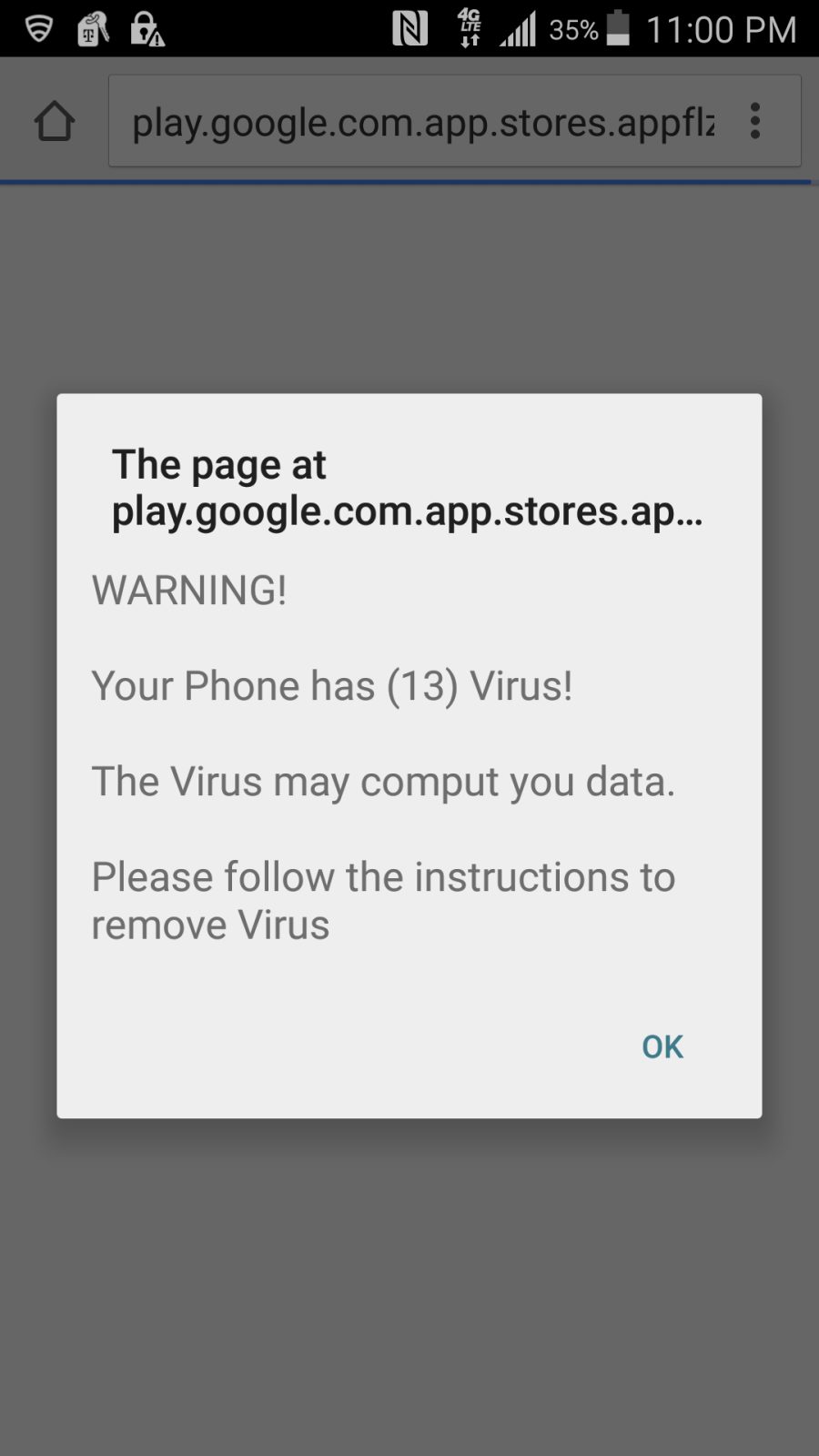This image depicts a smartphone screen displaying a suspicious webpage designed to deceive the user into thinking their device is infected with viruses. 

At the top of the screenshot, there is a black notification bar displaying various phone status icons including a '4G' symbol, signal bars, battery life at 35%, and the current time, 11:00 PM. Below the notification bar, the phone's interface shows a small 'home' symbol, followed by a partially visible URL, "play.google.com.app.stores.app.flz", which is truncated. Next to the URL, there are three vertical dots indicating a settings or menu option. A blue line runs below this section, serving as a separator.

The main content of the image is a phishing alert. It features a gray background with a prominent white dialog box. The dialog box header reads "The page at play.google.com.app.stores.ap..." The alert message in lighter gray text states, "Warning your phone has 13 virus." Notably, the word "compute" is misspelled. It should be "compromise." The message continues, "Please follow the instructions to remove virus." At the bottom right corner of the dialog box, there is a blue "OK" button likely intended to make the user proceed with potentially harmful actions.

The entire setup is evidently a fake alert, attempting to trick the user into believing their phone is compromised and coaxing them into taking unnecessary and potentially harmful actions.